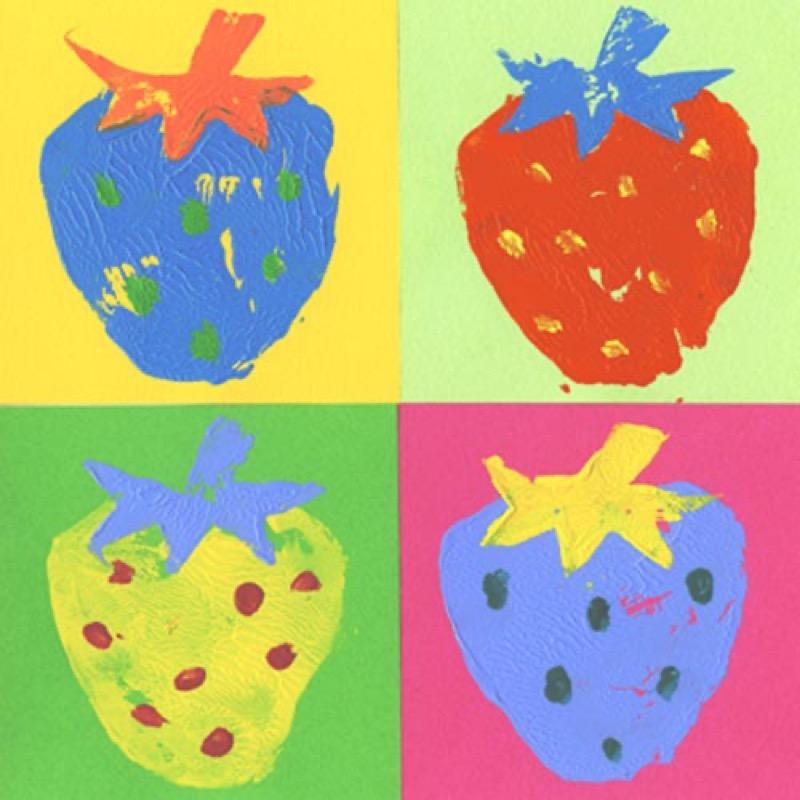This vibrant pop art painting features four distinct strawberries, each set against a unique background color, arranged in a square layout, divided equally into quadrants. The upper left quadrant showcases a blue strawberry with green seeds and an orange stem on a yellow background. Moving to the upper right, a red strawberry with yellow seeds and a blue stem stands out against a light green backdrop. The bottom left quadrant displays a yellow strawberry adorned with red seeds and a blue stem, set against a darker green background. Finally, the bottom right quadrant features a blue strawberry with dark green seeds and a yellow stem on a bright pink background. The painting, with its bold and contrasting colors, captures a whimsical and somewhat childlike quality, emphasizing the playful and energetic nature of pop art.